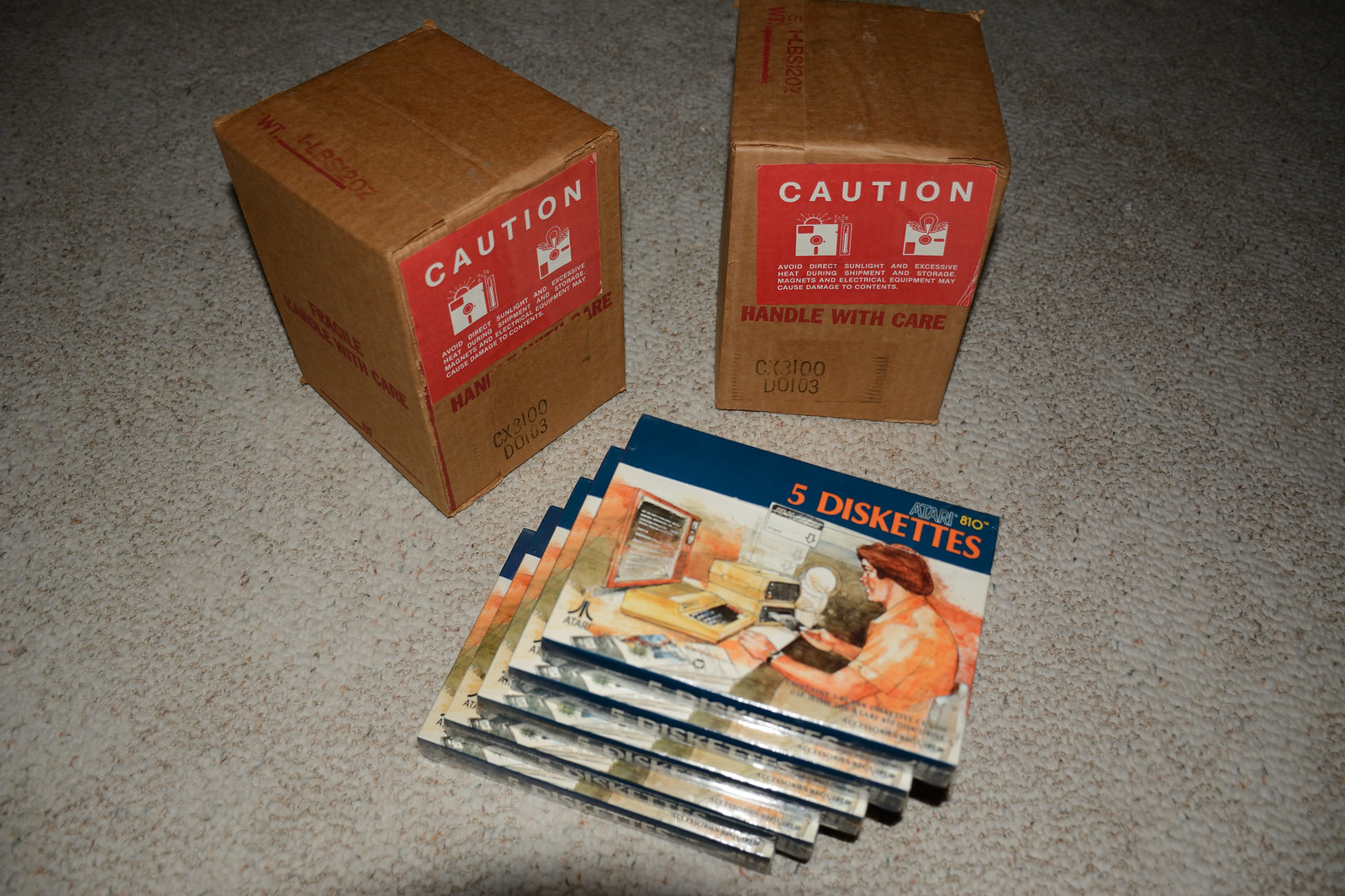This indoor color photograph captures a close-up view of a collection of vintage computer diskettes and accompanying cardboard boxes on a white, low-pile carpeted floor. Central to the image are five diskette cases featuring a drawing of a man in profile, inserting a diskette into an old computer drive with an old-style computer and printer on the desk before him. The top of each packet displays a blue rectangle with the words "five diskettes" in orange lettering. Surrounding these cases, in the top left and right corners of the image, are two brown rectangular cardboard boxes. Each box bears a red rectangular caution label with the word "CAUTION" in white text and a warning to "handle with care" underneath, albeit partially torn on the right box. The carpet, interspersed with brown and black speckles, provides a backdrop that emphasizes the vintage nature of these seemingly new but old diskettes designed for an Atari computer system.